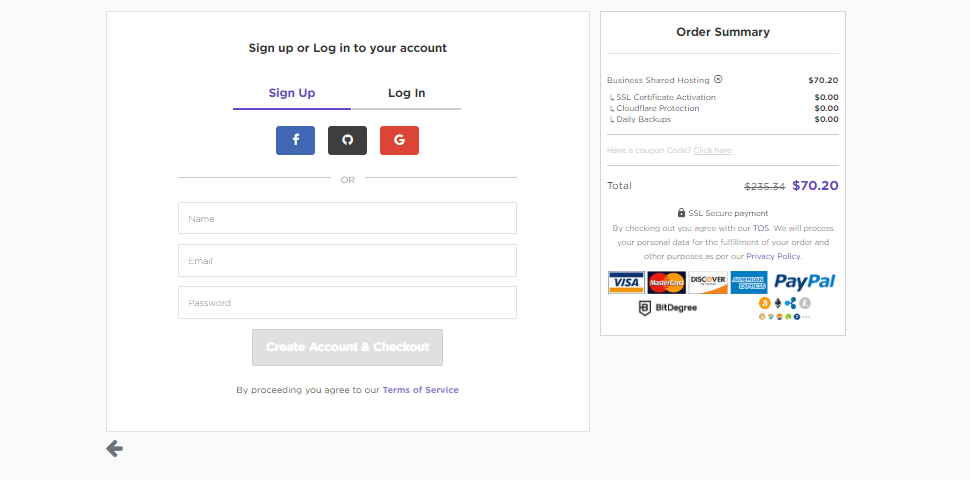The image depicts a payment page within an app, prompting users to either sign up or log in to proceed with their purchase. At the top of the page, there are two tabs labeled "Sign Up" and "Log In." Under the "Sign Up" section, various icons are displayed, allowing for registration through multiple platforms: an "F" icon for Facebook, an Apple logo for Apple ID, and a "G" icon for Google. Below these icons, users are prompted to input their name and other necessary details, followed by a "Create Account" button to finalize the registration and proceed to checkout. 

On the right side of the page, the "Order Summary" is displayed, indicating the total cost of the items in the cart as $70.20. Accepted payment methods include Visa, MasterCard, Discover, American Express, and PayPal. Users must complete the sign-up process and provide the shipping information to finalize their purchase and determine the delivery destination.